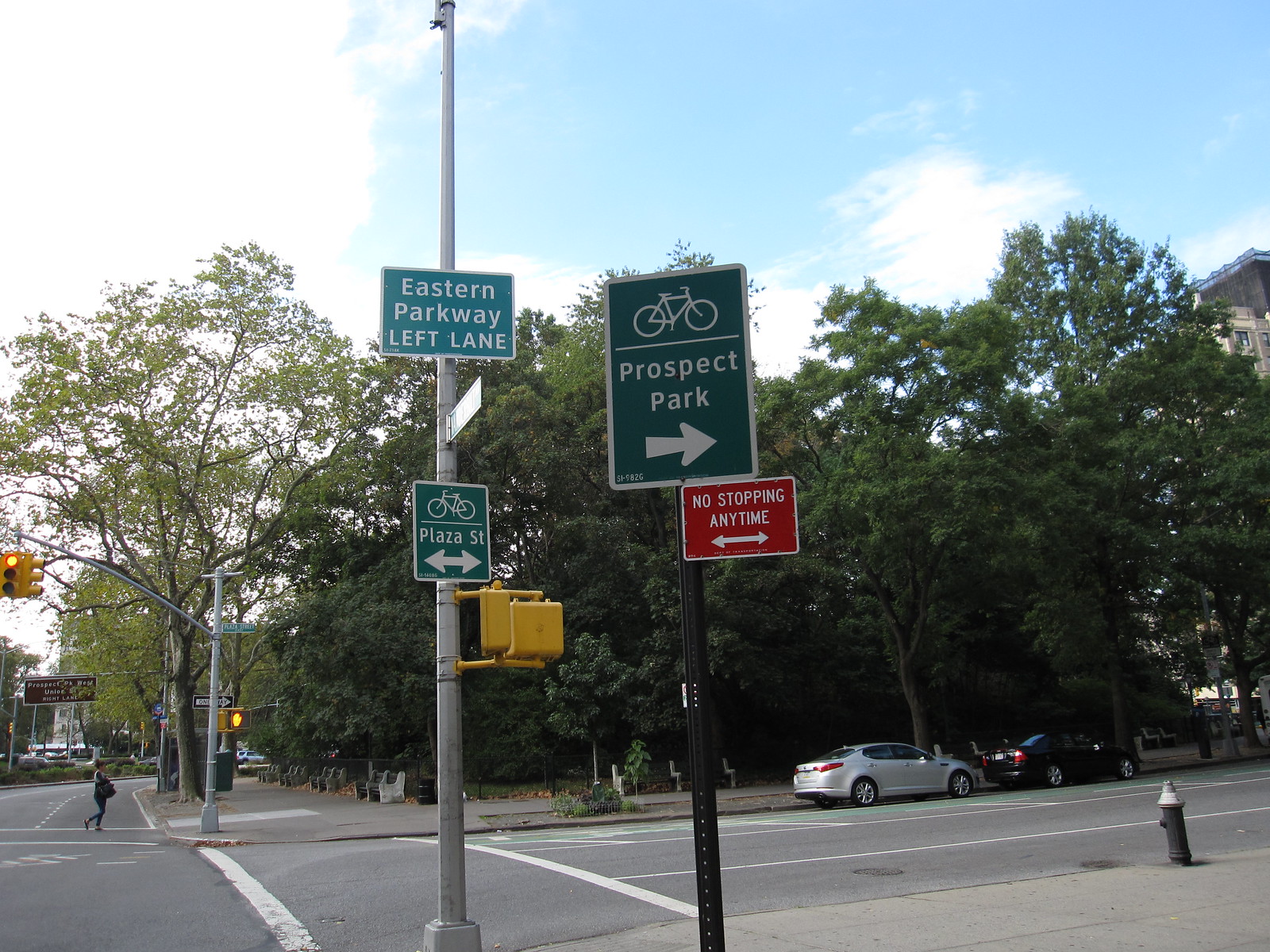In this detailed photograph of a bustling city street corner, the intersection of Eastern Parkway and Plaza Street is vividly captured. Prominent street signs on a light pole indicate directions to Prospect Park, with additional notifications for bike routes and a 'No Stopping Anytime' warning in red. A nearby traffic signal glows red as a woman with short or long sleeves, suggesting moderate weather, crosses the street via the crosswalk. The street is flanked by numerous green trees and features a gray fire hydrant on the corner. Two cars—a gray one and a black one—are parked along the curb. To the right, the edge of the frame hints at a building or structure. The overall ambiance is bright, though the sky is a mix of blue and gray hues, adding to the serene yet active urban scene.